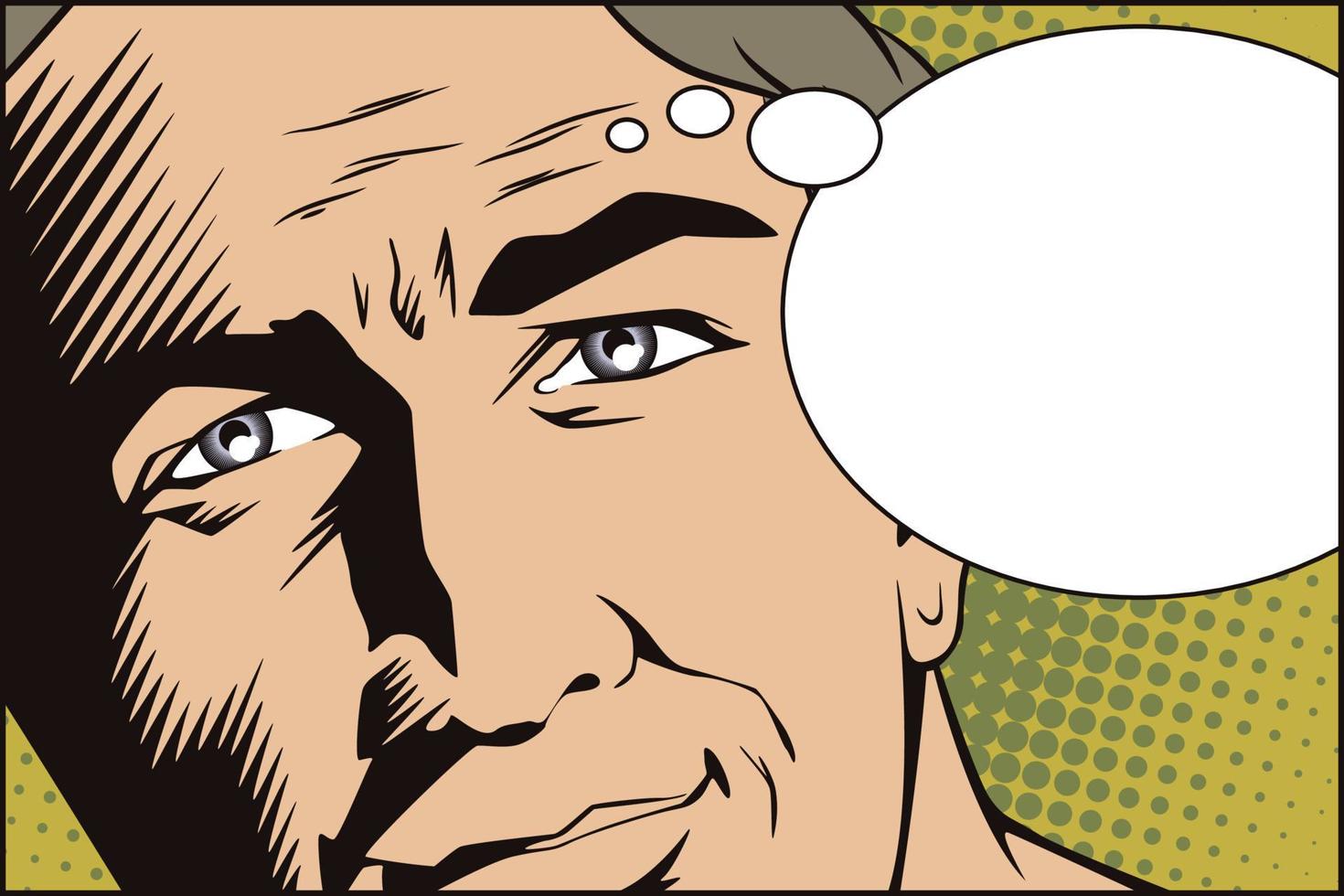This comic-style image features a close-up of a light-skinned man's face, primarily positioned to the left side of the panel. The man has wavy, light brown hair with hints of gray and distinguished black eyebrows. His silver-gray eyes are accentuated by visible wrinkles on his forehead and the pronounced shading on the right side of his face, which also extends to his right nostril. The image employs strong black lines to outline the man's features, imparting a sense of strength and shadow across his visage. A blank thought bubble emerges from above his left eyebrow, indicating contemplation without any text. The background is a vivid yellow adorned with olive green dots that vary in size, clustering more densely towards the edges and creating a dotted gradient effect that frames his face, further enhancing the comic book aesthetic.